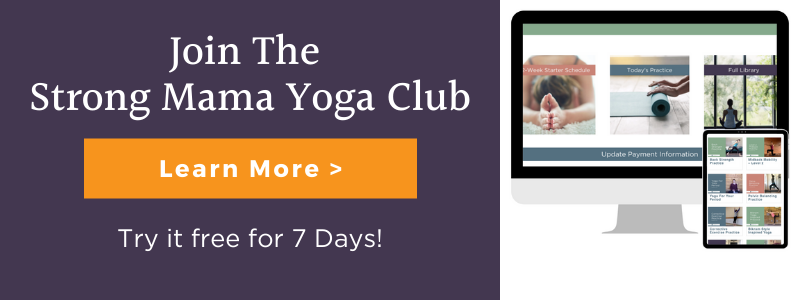In this detailed image of a web design, a sleek MacBook occupies the right side of the frame. Beneath it, an iPad displays an individual in a yoga pose, emphasizing calm and focus. The desktop screen exhibits well-organized text that reads: "Week Starter Schedule," "Today's Practice," "Full Library," and "Update Payment Information." On the left side of the image, prominently featured text invites the viewer to "Join the Strong Mama Yoga Club." Additional enticing details include "Learn More" and an offer to "Try it for free for seven days," encouraging engagement and exploration of the yoga club. The overall design is clean, modern, and inviting, effectively promoting the yoga club and its online resources.